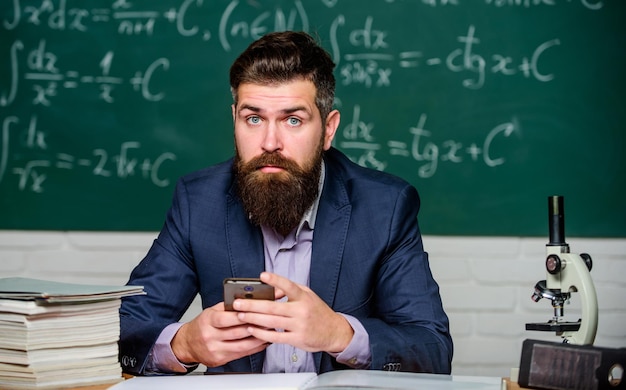The photograph depicts a young Caucasian man, likely a professor, seated behind a desk in an indoor setting. He has bright blue eyes and neatly combed dark brown hair slicked back. His full, shiny, dark brown beard and mustache are meticulously groomed. He wears a shiny blue blazer over a light purplish-blue collared shirt. The man is captured from about the solar plexus up, with his elbows resting on the desk and his hands holding a cell phone. His raised eyebrows and direct gaze at the camera suggest he may have just been interrupted.

The desk in front of him holds an open book, a stack of papers to his left, and a white microscope to his right. The background consists of a white-painted brick wall on the lower half, and a green chalkboard on the upper half, covered with white chalk equations including geometric formulas such as "dz over 52 squared equals ctg times x plus c." The photograph is a small rectangle, approximately five inches wide and three inches high, capturing the scene in a detailed yet intimate manner.